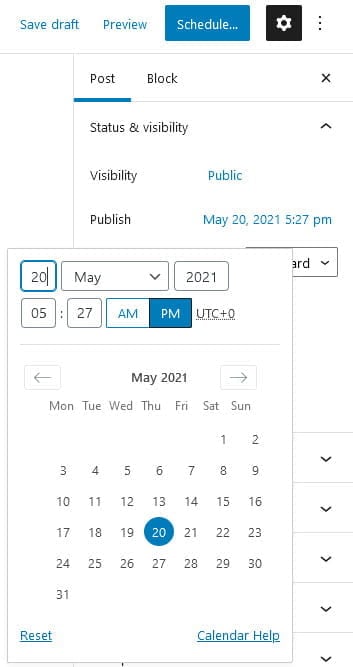The image showcases a detailed schedule interface. In the top left corner, it begins with the "Save Draft" option. To its right, there is the "Preview" option, followed by the "Schedule" button, which is highlighted in a blue box. Further right, we find a white gear icon enclosed in a black box, and to the far right, there are three vertical dots indicating additional options.

Below this row, the interface is divided into two main tabs: "Post" and "Block," with "Post" being selected, indicated by a blue underline. Under the "Post" tab, there is a section titled "Status and Visibility," which is expanded to reveal two specific options. The "Visibility" is set to "Public," and the "Publish" option is scheduled for May 20th, 2021, at 5:27 PM.

Further below, a pop-up calendar window is displayed, specifically highlighting May 20th, and indicating the selected time as 5:27 PM.